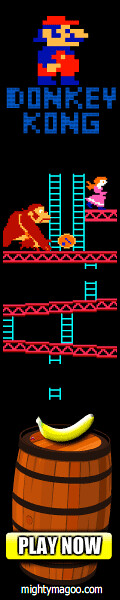The advertisement is a tall, vertical banner likely from a website, promoting the classic video game Donkey Kong. The background is predominantly black, creating a striking contrast. At the top, the title "Donkey Kong" in a bold, blue retro font captures immediate attention, accompanied by a character resembling Mario from Super Mario Brothers, dressed in a red hat, red overalls, a blue shirt, blue shoes, and sporting a blue mustache. Below the title, the classic Donkey Kong playing field is depicted, featuring red girders and green ladders. Donkey Kong himself is perched at the top, releasing a barrel, while the princess stands just slightly higher to the right in a pink dress with yellow hair. Toward the bottom of the ad, a detailed drawing of a wooden barrel with dark brown straps is shown, topped with a yellow banana. A yellow rectangle overlay with white capital letters reading "PLAY NOW" invites action, and at the very bottom, the website "MightyMagoo.com" is prominently displayed in white font.